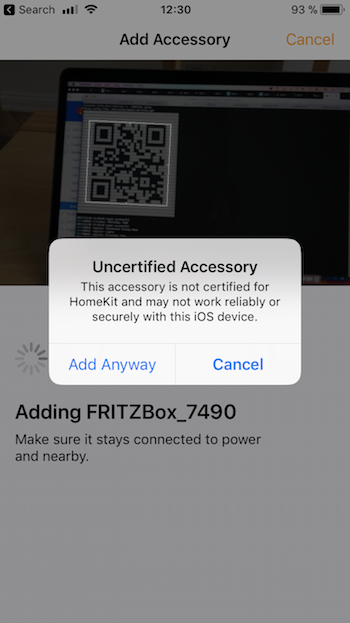This image is a screenshot taken from an iPhone, displaying an Apple HomeKit accessory screen with a prominent pop-up box. The background of the screen is white, creating a clean, focused view. 

In the center, a pop-up notification box titled "Uncertified Accessory" warns that the accessory is not certified for HomeKit and may not work reliably or securely with the iOS device. Within the pop-up, there's an option to "Add Anyway" in blue text, and to the right, "Cancel" in bold blue text.

In the background, at the top of the screen, the heading "Add Accessory" is centered, with "Cancel" displayed in small yellow text to its right. Below this heading, an image shows someone taking a picture of a QR code on a laptop, indicating the setup process. The rest of the background is white with minimal distractions.

To the bottom left of the pop-up box, a gray spinning icon indicates a loading or processing action. Below this icon, the screen displays "Adding Fritz Box_7490" in large, bold font. Directly underneath in smaller text, it advises users to "Make sure it stays connected to power and nearby,” providing essential instructions for the setup process.